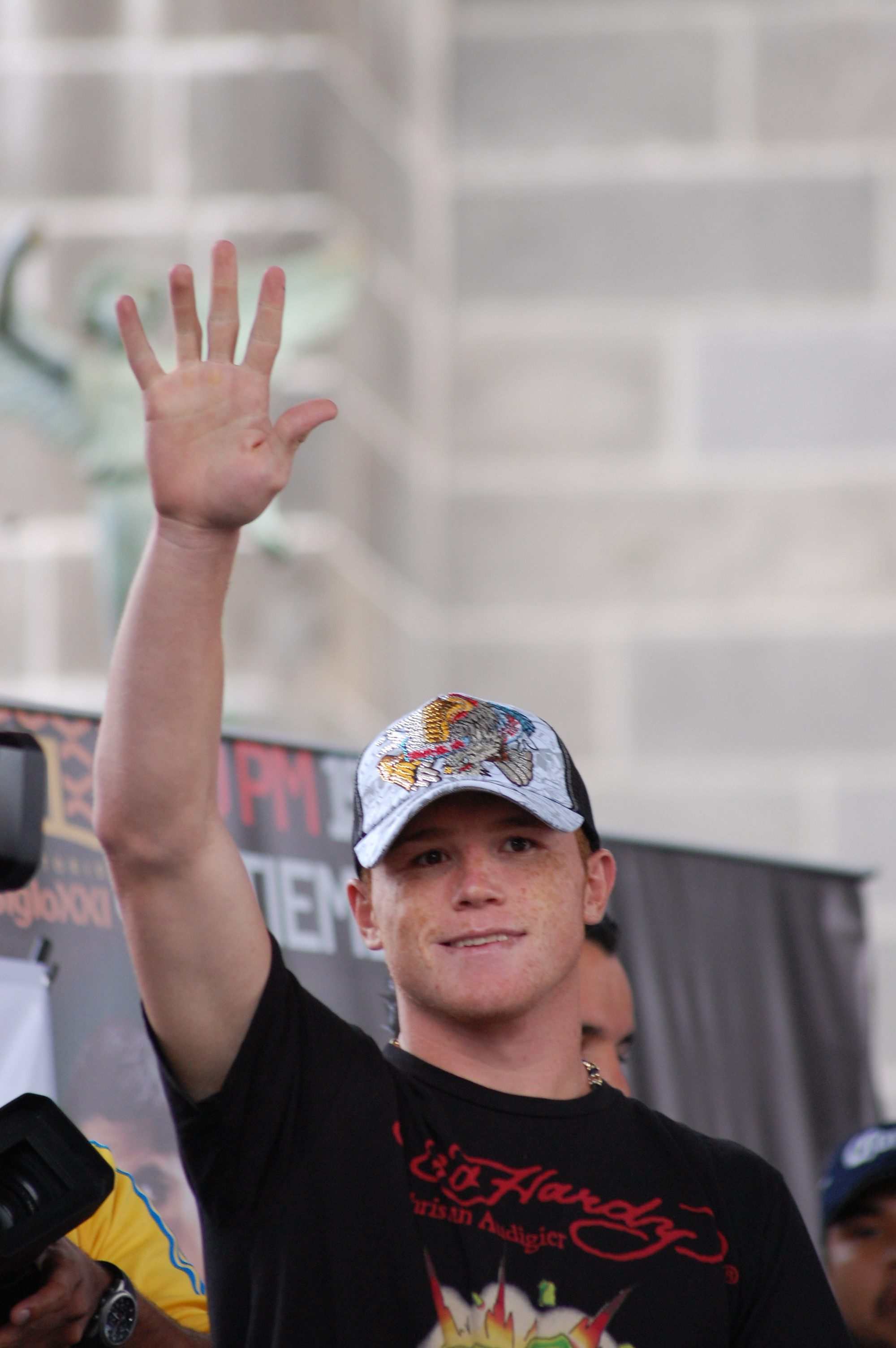In this image, a man wearing an Ed Hardy hat stands prominently at the center, waving towards a crowd. Behind him, a tall brick wall stretches across the upper part of the scene, adorned with some indistinct posters and signs. Scattered on either side of the man are several people handling camera and filming equipment, suggesting that an event is taking place. The overall setting remains ambiguous, potentially indoors or outdoors, but the bustling atmosphere hints at a lively gathering. The color palette includes shades of gray, white, green, yellow, blue, red, and black, adding to the vibrant feel of the scene.